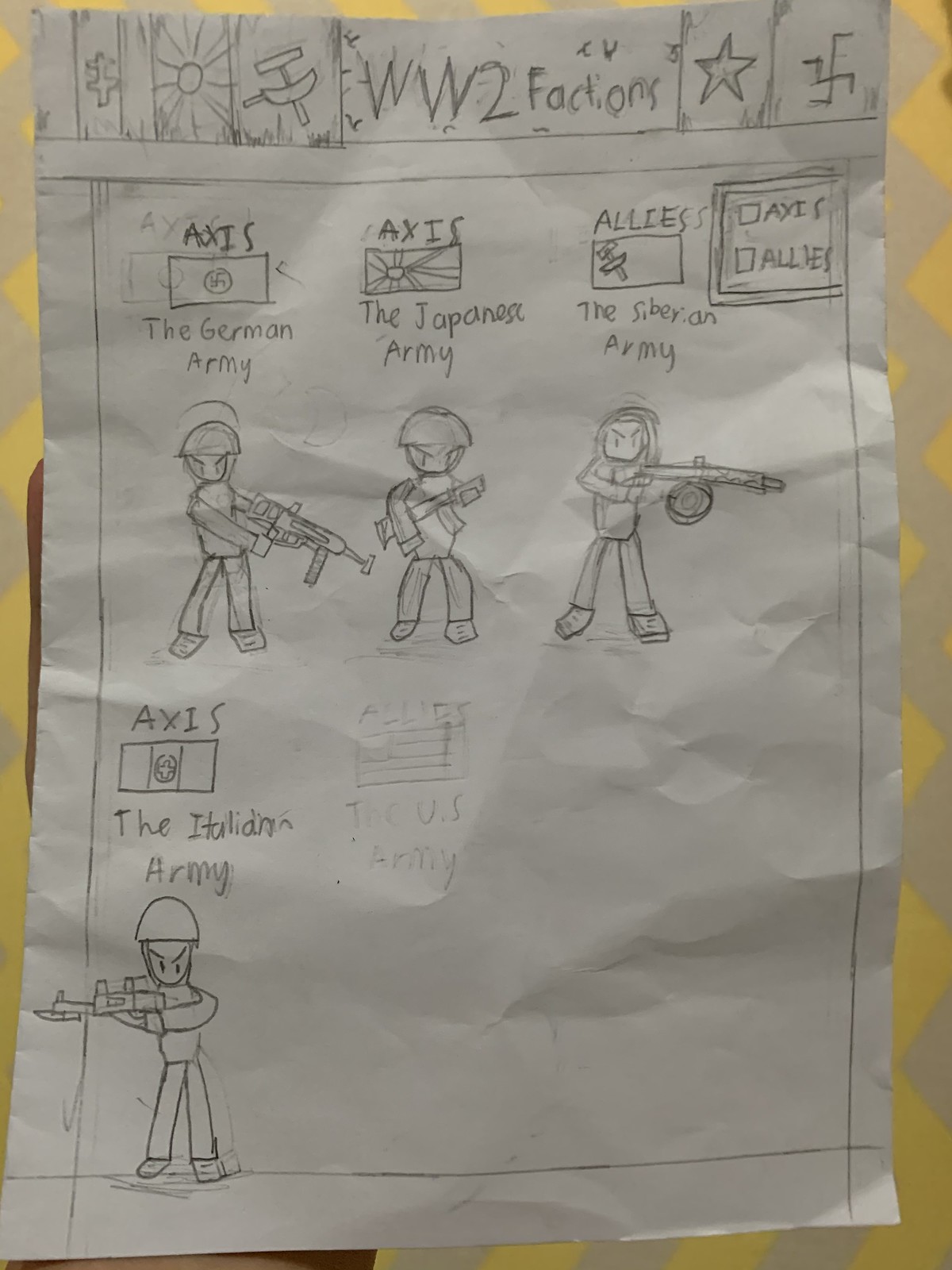This is a detailed pencil drawing on a white piece of paper depicting various World War II factions. At the top center, it features the title "WW2 Factions." To the left of the title, there are small squares, while the right side showcases a sun and several other symbols, including a star and a swastika. The bottom section of the page illustrates soldiers from different armies, labeled as "Axis and Allies." Specifically, it portrays the German Army, Japanese Army, Siberian Army, and Italian Army. There was also a depiction of the U.S. Army, although it has been erased. The soldiers are intricately drawn, each holding guns and wearing hard hats.